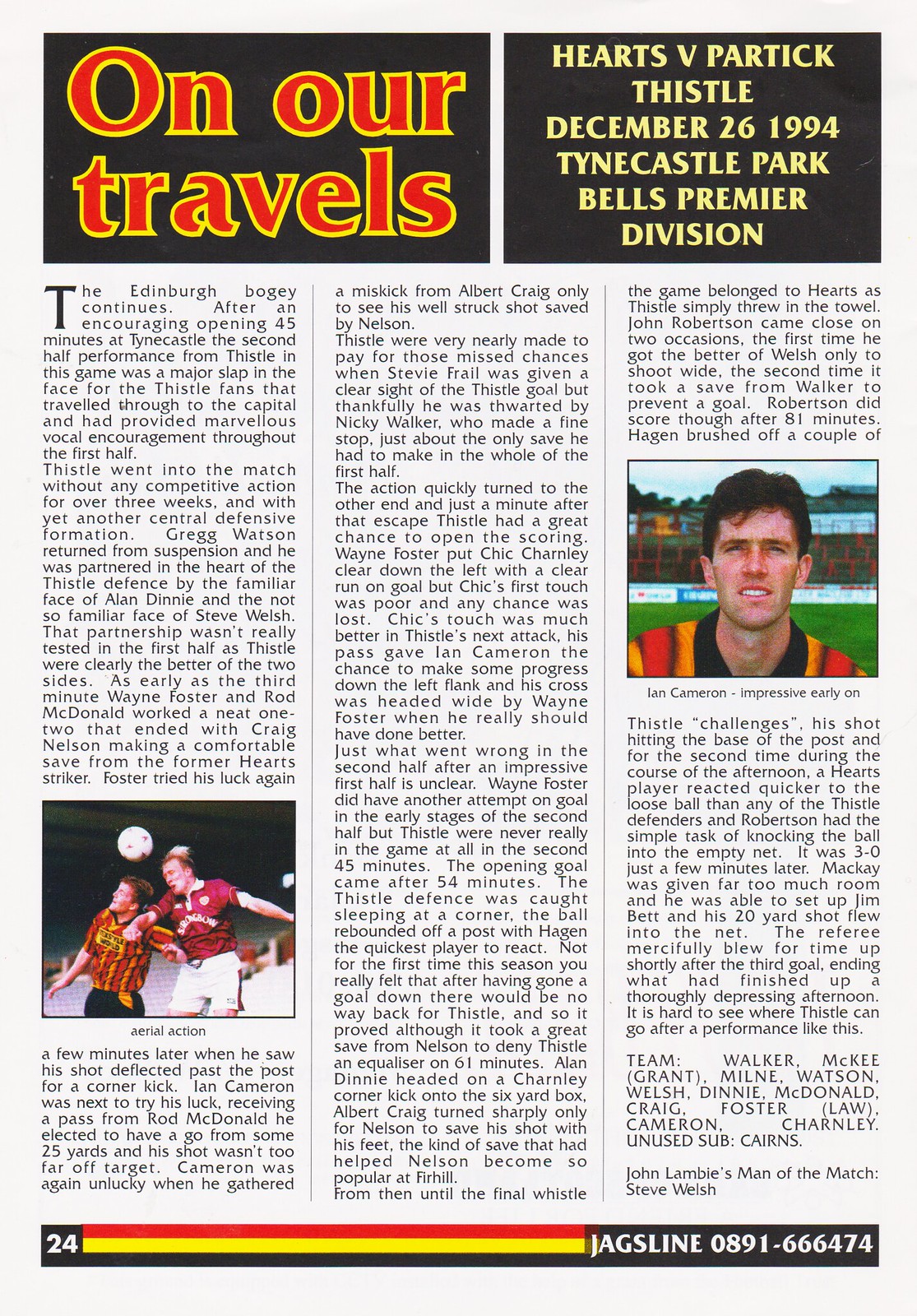This image depicts a page from an old sports magazine, likely from a soccer-focused issue. The page measures approximately six inches tall by four inches wide and is dominated by a lengthy three-column article printed in extremely fine text. At the top of the page, there are two large black rectangular banners. The left banner features the title "On Our Travels" in red text with a yellow outline, while the right banner displays the matchup "Hearts vs. Partick Thistle, December 26, 1994, Tyne Castle Park, Bells Premier Division" in yellow text. 

In the left column towards the bottom, there is a color photograph captioned "Aerial Action." This image shows two soccer players of Caucasian descent, airborne with their arms outstretched, vying for a header. One player wears a red short-sleeved shirt with white shorts, while the other sports a yellow and orange vertical striped shirt with black shorts. The soccer ball hovers just above their heads, highlighting a dynamic moment in the game.

The right column features another color image, this time of Ian Cameron, identified by the caption "Impressive early on." Cameron, a man of Caucasian descent with short brown hair, is depicted wearing a gold and red striped shirt. Below this photo, at the very bottom right corner of the article, there is a list labeled "Team" which includes players named Walker, McKee, Grant, Milney, Watson, Welsh, Dinney, McDonald, Craig, Foster, Law, Cameron, Charnley, along with unused substitutes Cairns and John Lambles. It also notes Steve Welsh as "Man of the March."

The lower part of the page features a black banner with a red and gold stripe containing the page number "24" on the left and the text "Jags line 0891-666-474" on the right, indicating a contact line presumably related to the Partick Thistle team.